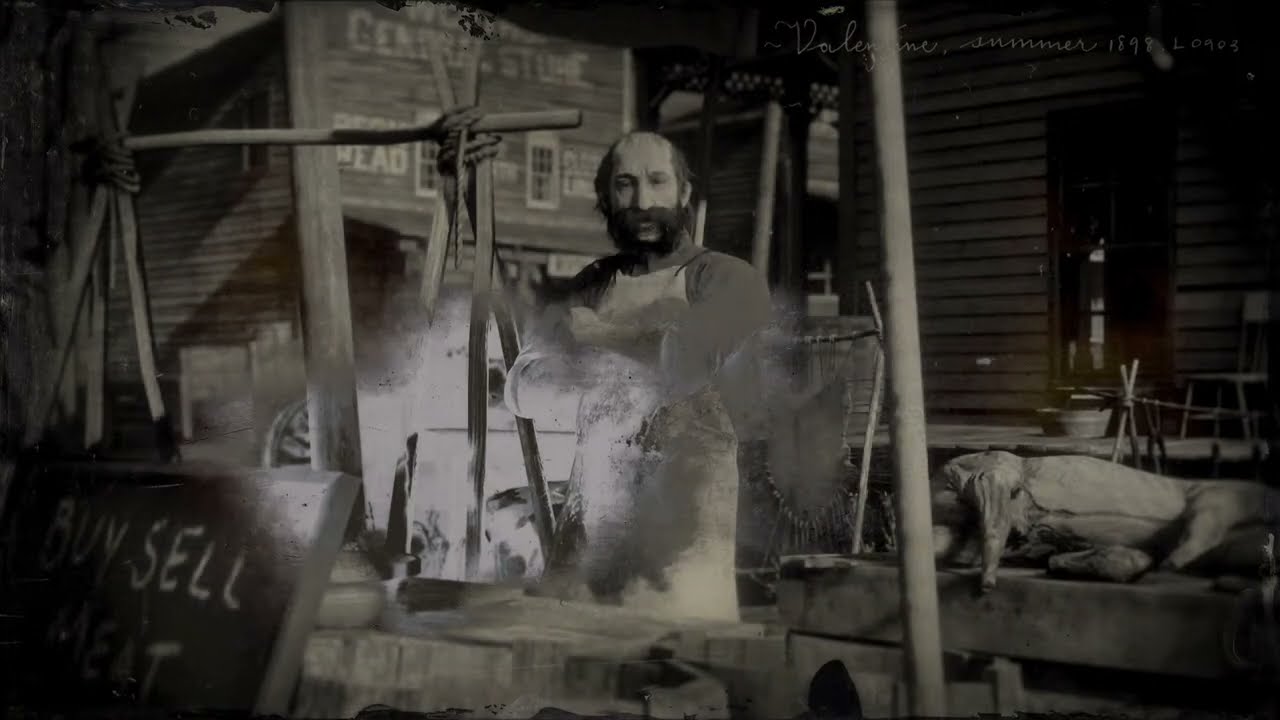This black and white (with a tint of brown) 3D image depicts a stern-looking man standing outside older wooden buildings reminiscent of an old western town. The man, appearing middle-aged with a balding head, dark eyebrows, and a full mustache and beard, dons a full apron that extends from his shoulders to beyond his knees. His hands appear to be over a fire pit, with smoke and a lit object suggesting he might be a glass blower or a butcher. His face shows signs of age, including wrinkles and a distinctive crease above his left eye.

To his right, a wooden structure composed of interconnected wooden rods and dowels is secured with rope. Nearby, there is a rectangular sign partially cropped in the lower left corner, displaying the words "buy" and "sell." Behind the man, wooden buildings form the background, one of which has a sign reading "General Store" above two windows. The upper part of the image features cursive writing with the word "summer" and a barely legible year, possibly "1899." A dead pig lies on a porch to the right side of the image, suggesting the man might be preparing to butcher it. Various tools and a stone table with an elephant-shaped object are also visible, contributing to the ambiance of a rustic, possibly commercial setting.